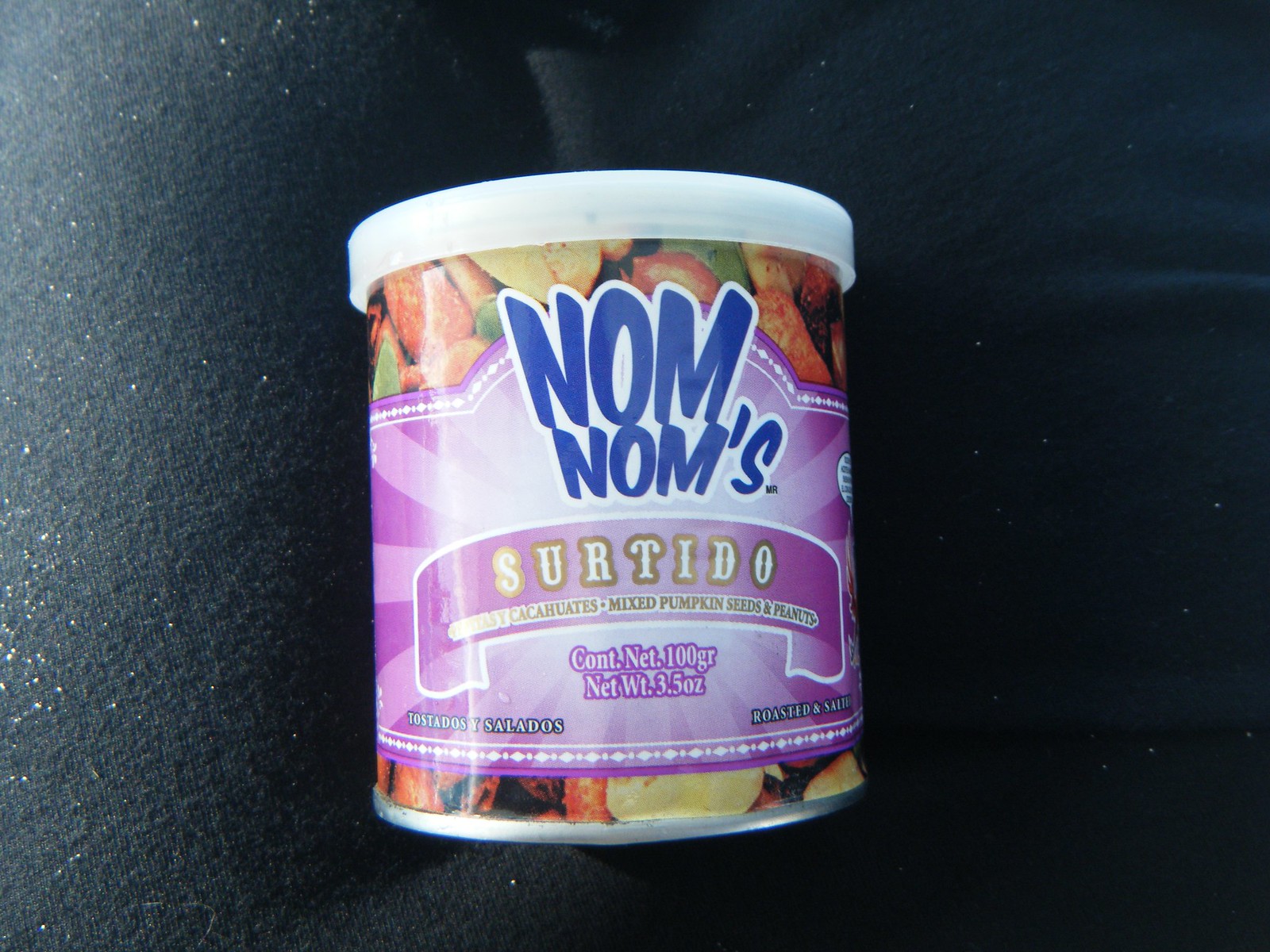The image is a photograph of a cylindrical cardboard tin of mixed pumpkin seeds and peanuts, branded as "Nom Noms." The tin rests against a soft black fabric, possibly someone's lap. The container features a white plastic lid that snaps onto the top. Dominating the design, the large, blue, all-caps "Nom Noms" logo with a white outline stands prominently at the top of the label. The label's primary color is a gradient of light to dark purple with radiant stripes. Below the brand name, the label reads "Sir T-Dough" and "mixed pumpkin seeds and peanuts," indicating the contents. The background of the label is adorned with images of roasted vegetables, highlighting the mix's ingredients. Additionally, the bottom of the tin specifies that the contents are "roasted and salted," with a Spanish translation, "tostados y salados," adjacent to it. The net weight is clearly marked as 100 grams or 3.5 ounces.